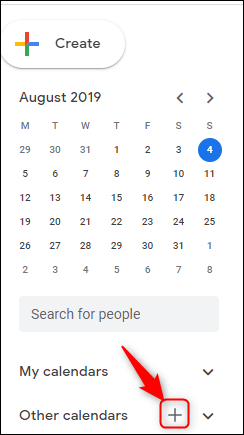This detailed screenshot captures a segment of a calendar from a mobile application interface. The image is enclosed by a thin black border with distinct right-angled corners. At the very top, the design includes a thin light gray line sitting below a narrow white stripe, followed by the primary white backdrop of the calendar page.

In the top left corner of the screenshot, there's a white pill-shaped button casting a subtle light gray shadow beneath it, with a multicolored plus symbol on its left side. The plus symbol is segmented with red on the top, orange on the left, blue on the right, and green on the bottom. To the right of the plus symbol, the button is labeled with the dark gray text "Create."

Just below, the text "August 2019" is centrally aligned in dark gray font. Flanking this text are gray navigation arrows, with the left arrow positioned to the immediate left and the right arrow to the immediate right, allowing users to switch between months.

The calendar grid starts with a row of abbreviations for the days of the week in gray text, arranged from left to right as M (Monday), T (Tuesday), W (Wednesday), T (Thursday), F (Friday), S (Saturday), and S (Sunday). Each column beneath these headers contains sequential dates, starting lightly with the numbers 29, 30, and 31 in the first row under M, T, and W respectively. These slightly lighter numbers indicate the overlapping days from the previous month. The days of August, displayed in black text, begin from 1 through 31, with the 31st falling under the first S (Saturday). Following the end of August, the numbers 1 through 8 of the subsequent month are again lightly printed. Notably, the date "4" is highlighted with a blue circle, emphasizing it as the current date within the calendar interface.

Below the calendar grid, there's a light gray search box featuring the placeholder text “Search for people” in dark gray. Beneath this search box, two lines of black text are spaced out. The first line reads "My calendars" followed by a space and a downward-pointing black arrow located on the right. The second line reads "Other calendars," maintaining the structural consistency of the drop-down menu.

This comprehensive description covers the detailed visual elements and layout specifics of the calendar screenshot, offering a clear and vivid depiction of the mobile application interface.